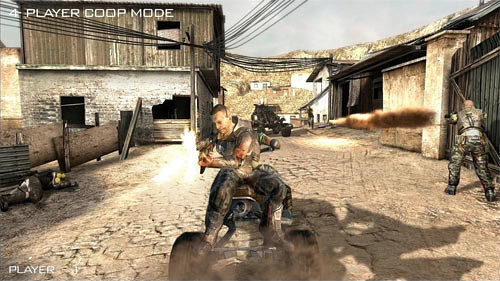In this detailed image from a first-person shooter video game, the scene is set in what appears to be the streets of an old, rugged city. The architecture consists of antiquated buildings, with one prominently on the left side of the image that features a wooden upper structure and a stone base, marred by a conspicuous hole from recent damage. The game interface displays "4 Player Co-op Mode" in the top corner and identifies "Player 1" in the bottom left corner.

On the right side of the image, more buildings line the street, maintaining the aged, sturdy aesthetic of the environment. Dominating the mid-ground, a vehicle seemingly advances toward the player's position, heightening the sense of imminent action.

A soldier clad in camo pants and a camouflaged top is visible on the right, armed with a gun and poised for combat. Directly in front of the player, atop a four-wheeler, another soldier is actively engaging, as evidenced by the visible muzzle flare from his weapon, suggesting a fierce and immediate firefight.